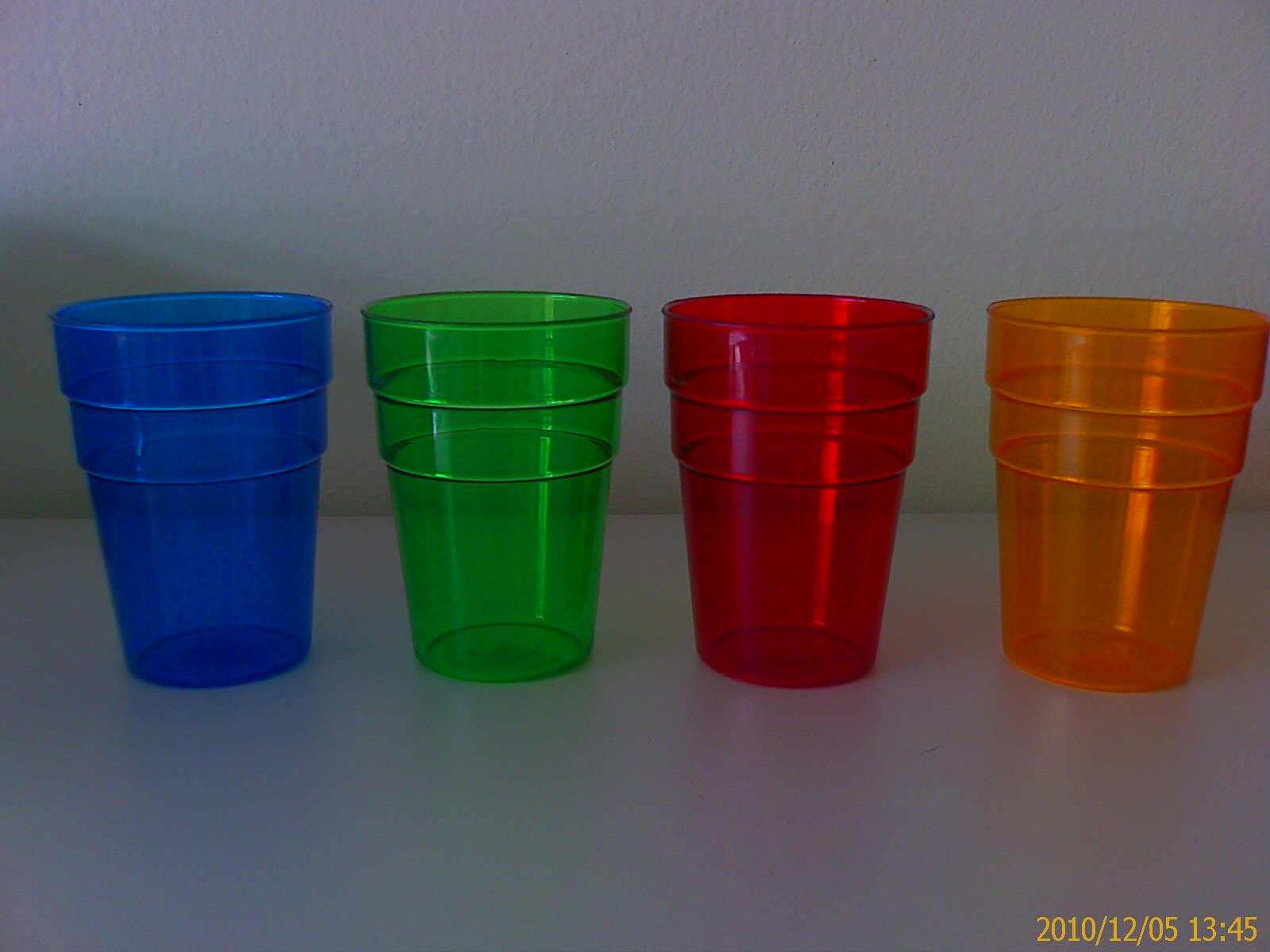The photograph, taken on December 5, 2010, at 13:45 (military time) as indicated by the yellow timestamp in the bottom right corner, captures four brightly colored, translucent plastic drinking cups arranged side by side on a flat, generic-looking white or off-white tabletop. The cups are positioned against a slightly textured white wall. Each cup, although empty, features a distinctive design with ridges toward the top and a thick outer band of plastic. From left to right, the cups are dark blue, green, red, and orange. They are translucent, allowing the colors to tint the background and cast shadows diagonally upward to the left, likely a result of a light source or camera flash, with noticeable reflections on the right-hand side of each cup except the blue one.